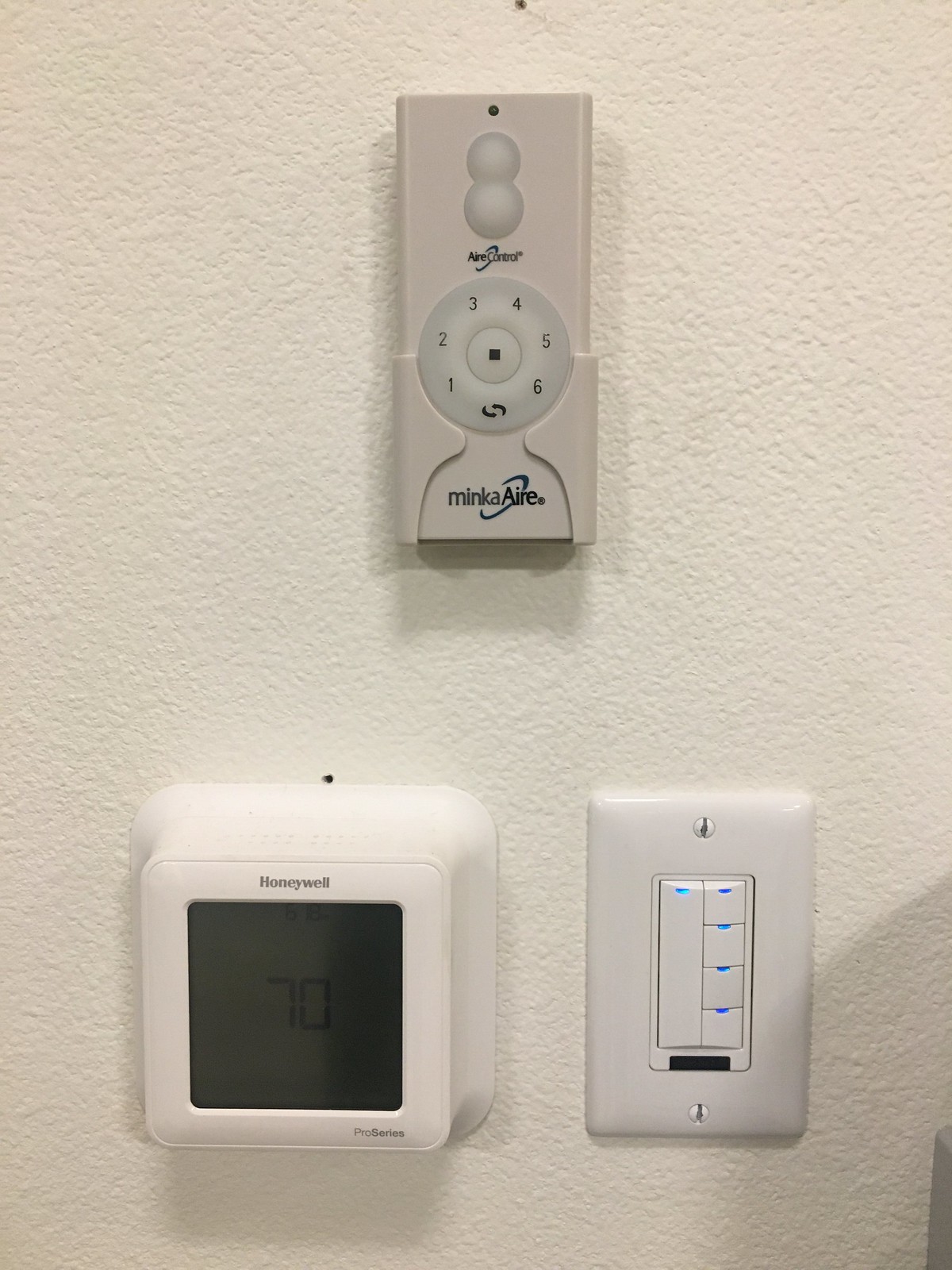A white wall features multiple devices: At the top is a rectangular Minka Air remote control. The remote is white and gray, with a dot near the top and a circular pattern resembling a snowman beneath it. Below the circles, the text "Air Controls" is visible followed by a numbered sequence (1 through 6) in gray. The brand name "Minka Air" is printed at the bottom, accompanied by a swirl logo. 

This remote is housed in a gray holder. On the lower part of the wall, the message "Honeywell" is visible on the left and "Pro Series" on the right, indicating the brand and series. A digital display reads "77." The whole unit encloses in a square plastic frame with sloped edges.

To the right of the unit is a switch panel: The left switch is a long rectangle with a small blue light at the top. To its right, there are four smaller square switches, each with a tiny blue light at the top. A black bar runs across the bottom of these switches.